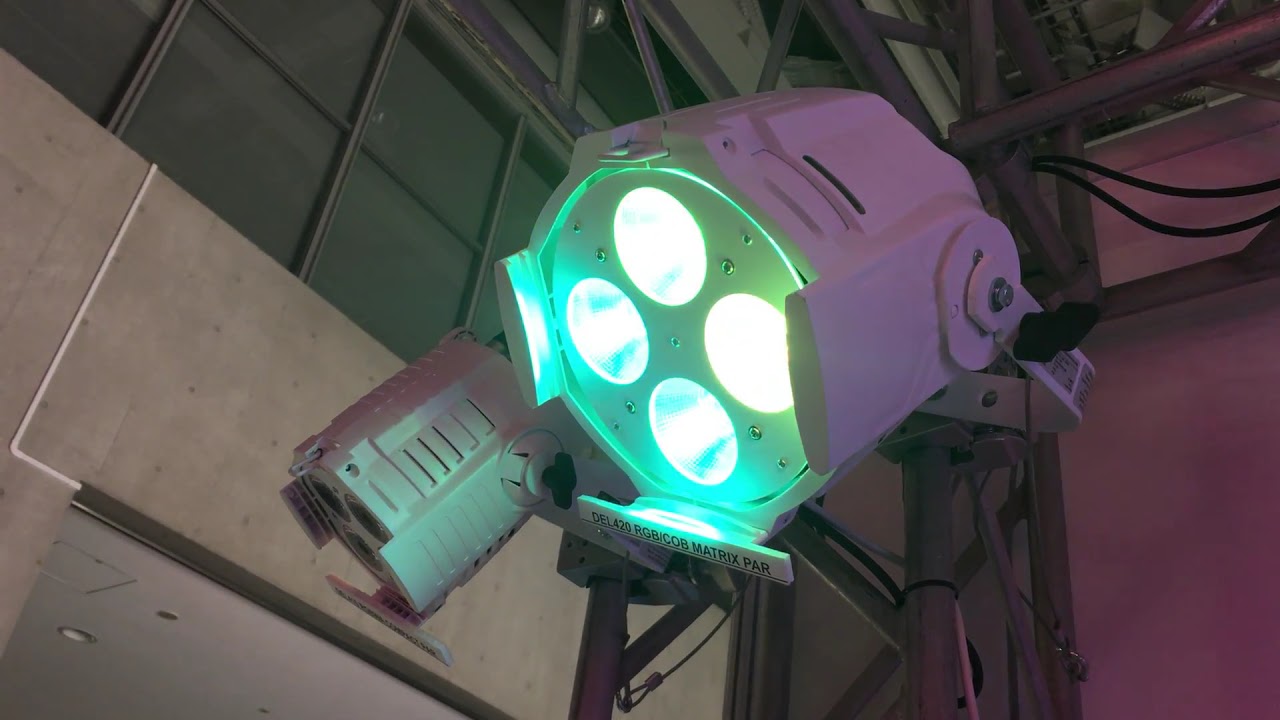The image captures an industrial recording studio ceiling scene, highlighting a section of intricate metal scaffolding adorned with two spotlights. The backdrop features a concrete wall halfway up, transitioning into square metal panels, with a visible small white PVC pipe running down a portion of the concrete. One spotlight, the focus of the image, showcases a circular design with four individual circular lenses on its face, emitting a gradient of greenish-blue and yellow light. This active light bears a small rectangular tag that reads "DEL420 RGB/COB Matrix PAR" in black capital letters. The second spotlight, mounted on the same metallic frame and pointed in another direction, remains off. The overall setting gives off a professional, yet stark industrial vibe, complete with the metallic complexity and robust structure of the scaffolding.